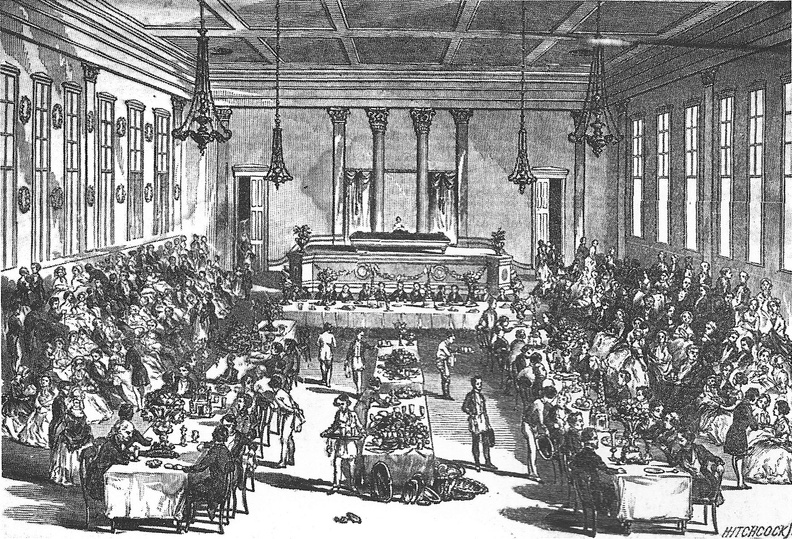The image is a highly detailed black and white lithograph depicting a Victorian banquet hall with an exceptionally tall, tent-like ceiling supported by ornamental pillars. At the far end of the hall, four central pillars seem to frame a stage or raised platform with a person seated at a desk, possibly indicating an important figure or event. In the foreground, tables are arranged in a U-shape filled with people engaged in lively conversation and enjoying a meal, while central tables appear laden with food, attended by servants. The high walls are adorned with numerous tall, rectangular windows, framed with intricate designs, allowing light to stream into the spacious hall. The scene is bustling, featuring a mix of elegantly dressed men and women, with many women in white, period-appropriate ball gowns. The room is filled with an air of festivity and social interaction, capturing a moment of historical gathering with stunning intricacy and depth.